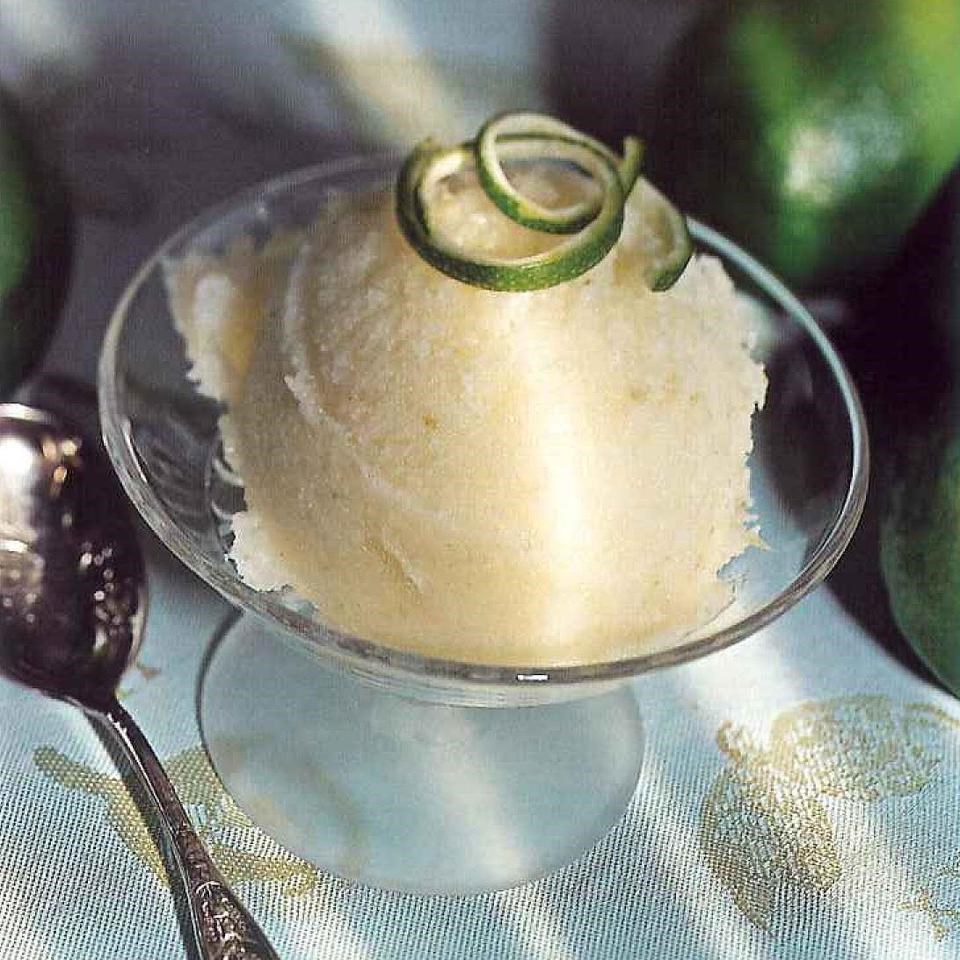In this photograph, there is a clear, bowl-shaped glass dish with angled sides, placed on a table setting. Inside the dish, a light yellow or golden, creamy-looking ball of shaved ice or sorbet is garnished with a spiral of dark green lime rind. The dish sits on a light blue tablecloth adorned with gold leaf designs. To the left of the dish is an intricately engraved silver spoon. The background features several dark green limes scattered around the table, with some visible on both the left and right sides of the image. The overall setup suggests a refreshing lime sorbet presentation, emphasized by the clear glass dish and elegant table setting.